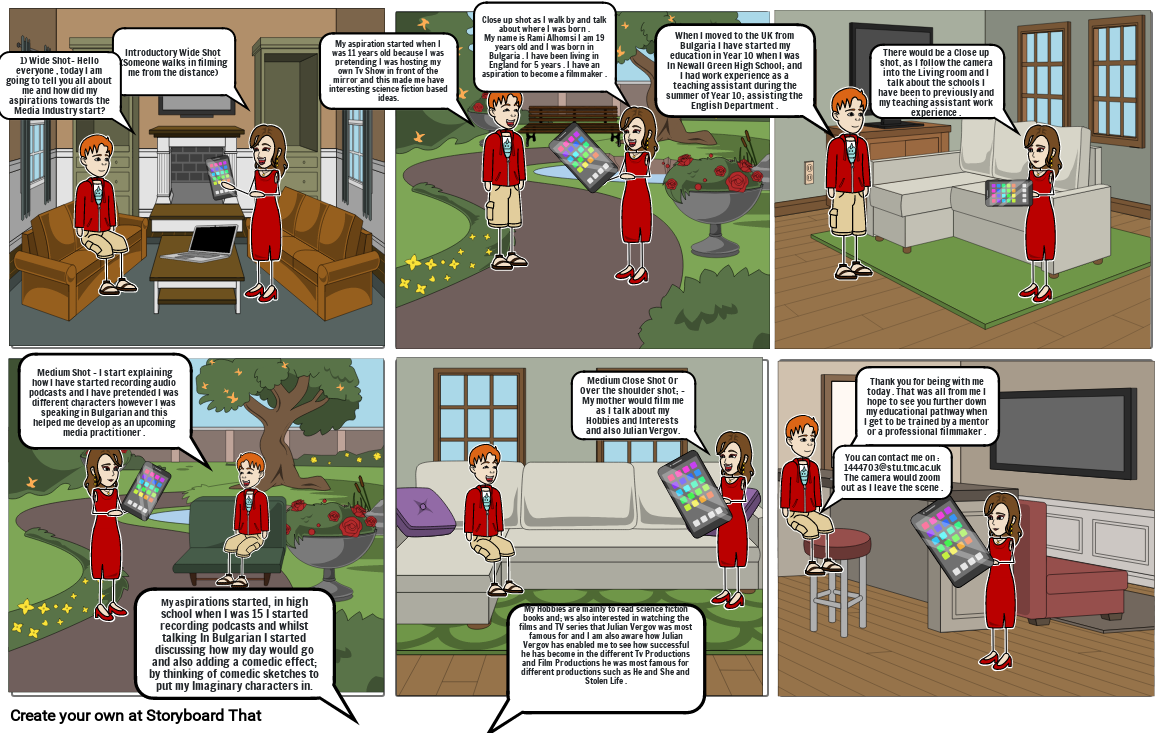This image promotes a storyboard screen composed of six panels, arranged in a grid with three on top and three on the bottom. Below the bottom left panel, there's black text that reads, "create your own at storyboard that," indicating it was created using an online tool. The storyboard features two characters prominently: a female dressed in a red dress and red pumps, holding a black tablet or video game device, and a male wearing a red jacket over khaki shorts and tennis shoes. They appear in various settings throughout the panels, each with speech bubbles that contain text too small to read clearly.

In the first panel, the characters are in a living room with white walls, brown couches, a gray floor, a silver laptop on a brown and white table, a TV on the wall, white cabinets, and a fireplace with white and gray bricks. The second panel depicts an outdoor park scene with green grass and trees, a gray pathway, a brown park bench, and flower pots containing red and yellow flowers. The third panel shows another living room scene with an L-shaped cream-colored sofa, a green rug, a brown wooden floor, a TV, and gray walls adorned with brown window frames.

The bottom row starts with the characters in another park-like setting where the male is sitting on a green bench and the female stands nearby. This scene includes the same feature of trees, bushes, and flowers as the previous park scene. The middle panel on the bottom row shows them in the living room with the cream-colored sofa and similar decor. The final panel presents them in a different room featuring a red sofa, a gray rug, a brown wooden floor, and a bar stool with a red seat and silver legs. In each panel, the female character holds her device, enhancing the continuity and theme of the storyboard.